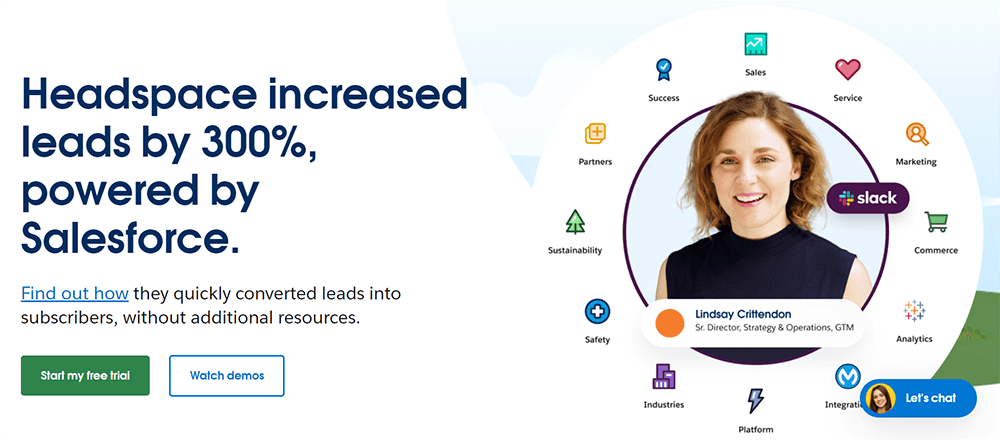This screenshot appears to be a segment of a website prominently featuring a success story about Headspace's achievements with Salesforce. On the left side, large dark blue text in four lines reads:

"Headspace increased leads by 300%
Powered by Salesforce"

Below this prominent statement, there's a clickable link that states "Find out how," detailing how Headspace effectively converted leads into subscribers without the need for additional resources. 

Further down are two buttons for user interaction: a green button labeled "Start my free trial" and a blue-outlined button labeled "Watch Demos."

To the right of the text, there's a circular image of a woman surrounded by 12 icons arranged in a clockwise manner. Each icon has an associated label, denoting different Salesforce features and benefits, which read as follows:
- Sales
- Service
- Marketing
- Commerce
- Analytics
- Integration
- Platform
- Industry
- Safety
- Sustainability
- Partners
- Success